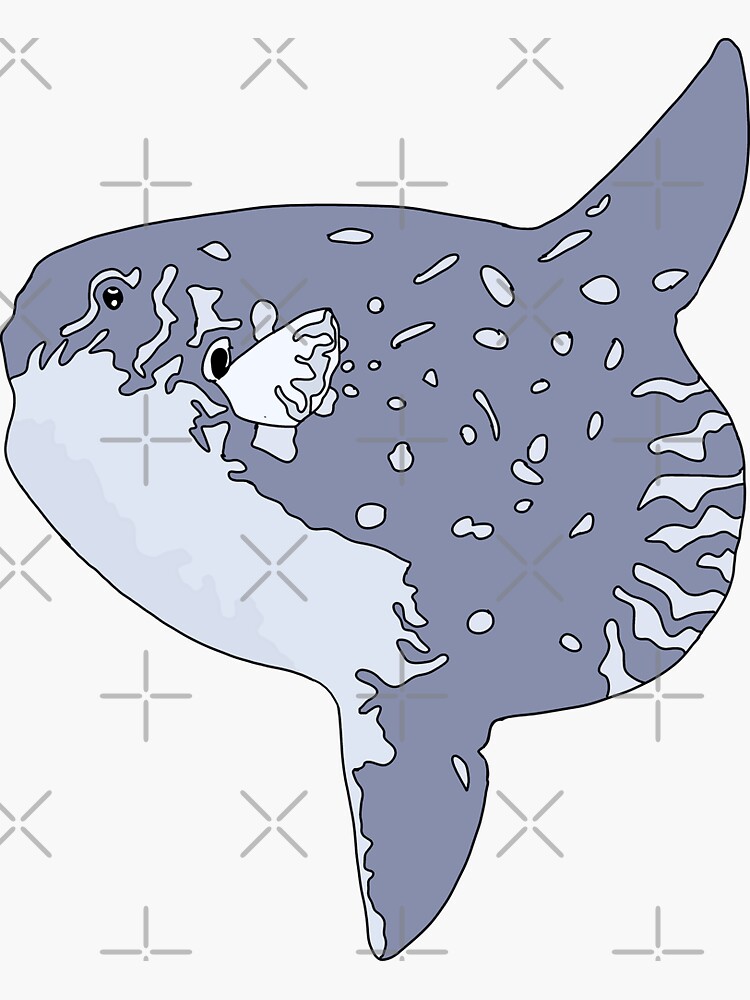This abstract illustration features a bluish-gray sea creature, perhaps a whale or shark, depicted on a white background with scattered gray markings, including crosses and X's. The animal boasts a large, robust body with a lighter blue underbelly. Its detailed skin showcases an array of patterns, such as unevenly shaped circles and distinct squiggly lines of a lighter shade. Noteworthy features include a dorsal fin positioned towards the right and a central ventral fin, with a small whitish fin near its right "eye," adorned with gray markings. The right side of its back displays seven short, uneven stripes of the lighter color, further enhancing the whimsical nature of this artwork. The creature's eyes are represented by black dots, adding to its enigmatic appearance in this captivating piece.